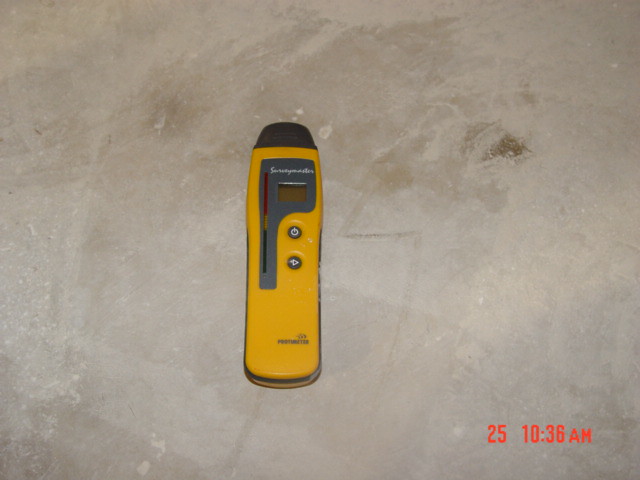This image showcases an unfamiliar narrow rectangular tool positioned on an off-white, beigeish concrete floor. The tool, primarily yellow with a dark gray top, features a rounded bottom. It includes several control elements: a gray central part with gray buttons and a long side stripe that transitions from green to red, resembling a temperature gauge. Additionally, there appears to be a display for readings and a possible power button underneath. Indistinct letters are visible on the device, yet they are illegible. In the bottom right corner of the image, an orange time stamp reads "25 10:36 AM." The concrete floor is marked with smudges or natural discolorations, creating various shades of beige and brown.